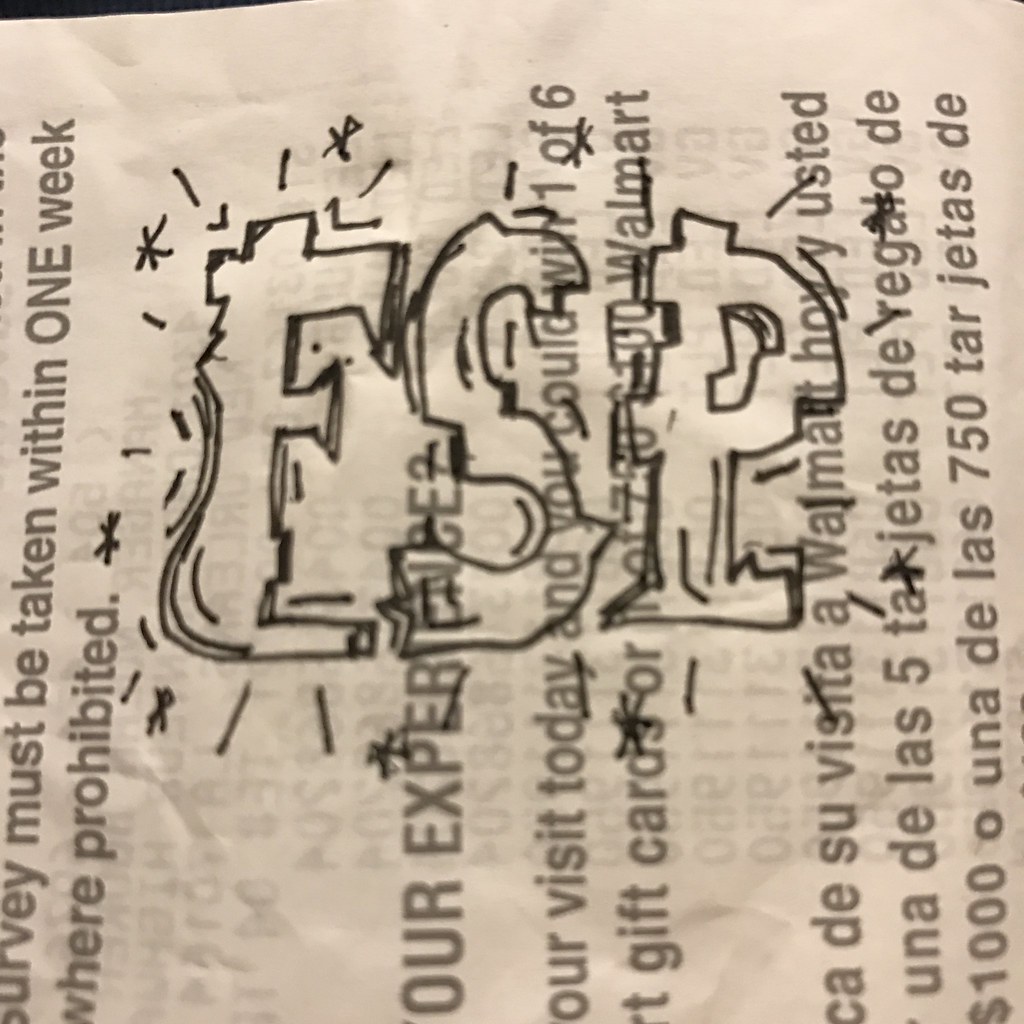This photograph captures the back of a Walmart receipt, oriented sideways against a black background. The receipt, colored grayish-white, shows faint, almost legible print bleeding through from the other side. In clear blackish-gray text, it reads, "Survey must be taken within one week where prohibited," followed by, "Our experience?" and, "Our visit today and you could win one of six $100 Walmart gift cards." Below, the same message is repeated in Spanish. On top of this text, someone has doodled in a graffiti style using black pen. The letters "ESP" are prominently featured in block, bubble-like letters, adorned with stars, dashed lines, and squiggles, adding a whimsical, modern touch to the receipt.